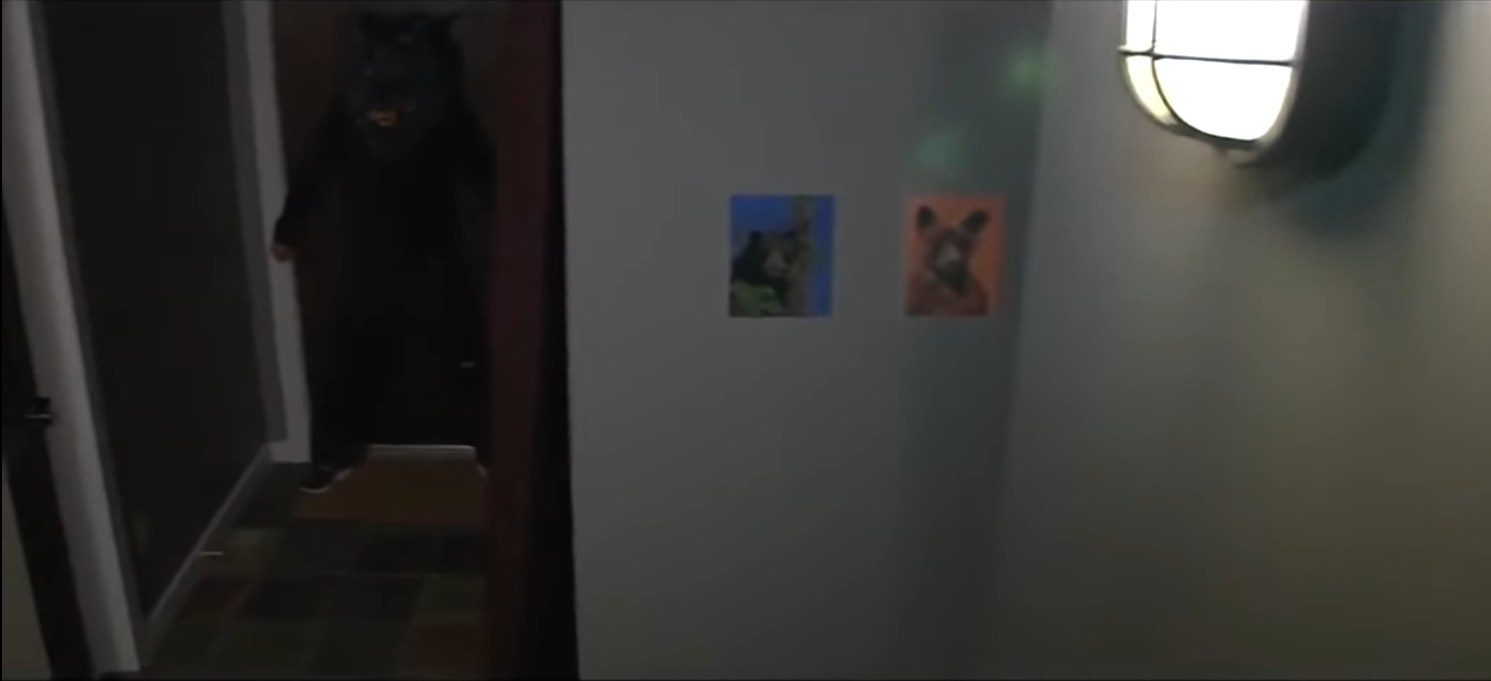In the image, we see a horizontal rectangular room with light gray walls. A light fixture is positioned near the top right corner, casting a noticeable glare. Two papers are affixed to the wall, each featuring blurry images of animals; the left one has a blue background, and the right one has a pink background. Above the pink paper, two green light reflections are visible, forming a diagonal pattern from the left ear of the animal to the top right corner. To the left of these papers, there is a brown door framed with white molding and a dark surface in between. Standing in the doorway is a person dressed in a dark animal costume, partially visible with their right sneaker and hand exposed. They are standing on a tan horizontal floor mat with the rest of the floor noticeable beyond the mat.